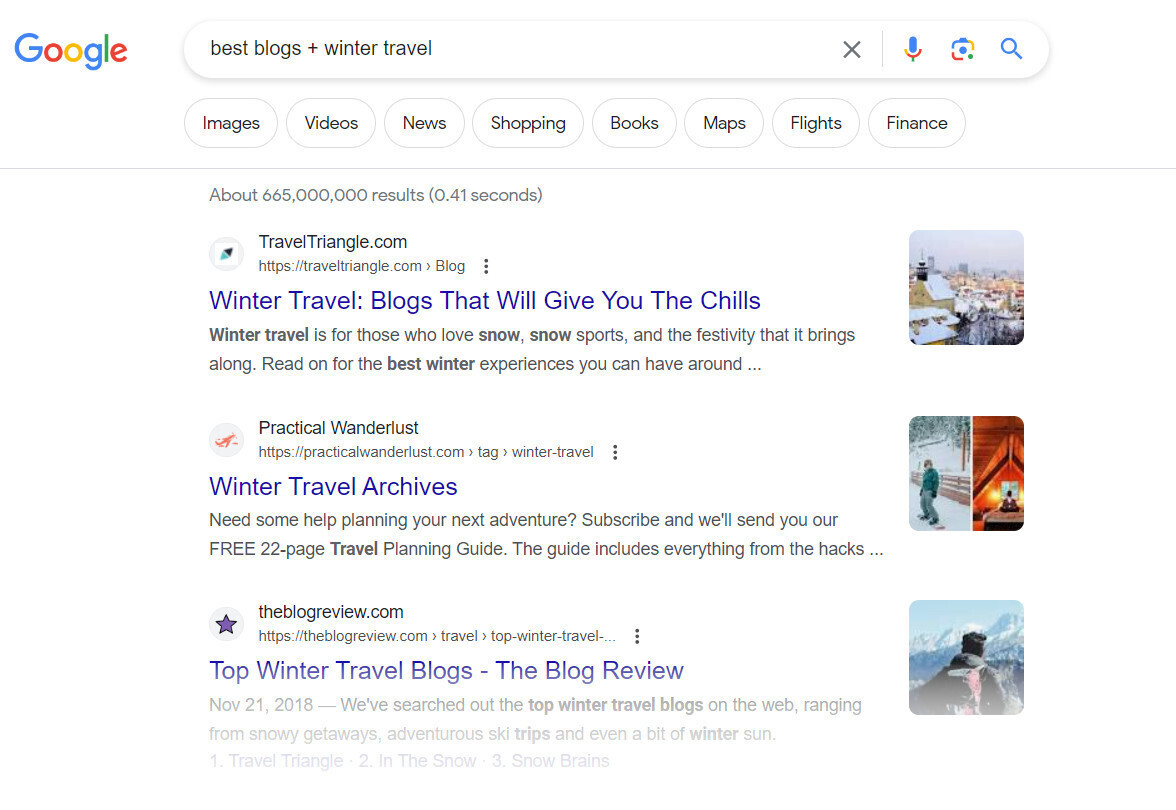In this image, we see the results page of a Google search query for "best blogs winter travel." The interface features the Google logo on the left and a search bar to the right containing the search terms. Adjacent to the search bar are icons including a gray 'X', a microphone, an image icon, and a blue magnifying glass. Below the search bar, there are eight categories displayed left to right: Images, Videos, News, Shopping, Books, Maps, Flights, and Finance. Further below, in gray text, it states "About 665,000,000 results (0.41 seconds)."

The top search result is from traveltriangle.com, titled in blue text: "Winter travel blogs that will give you the chills." Below it is a brief description. The second result is from practicalwanderlust.com, with the title "Winter Travel Archives" also in blue, followed by another descriptive sentence. The third result is from theblogreview.com with the title "Top Winter Travel Blogs - The Blog Review" displayed in blue text.

To the right of each search listing are images. The first result features an outdoor escape scene of a city in winter. The second result has two images: on the left, a snowboarder, and on the right, a plain orange background. The third result showcases a snowy mountain with a light blue sky. The entire layout is set against a white background.